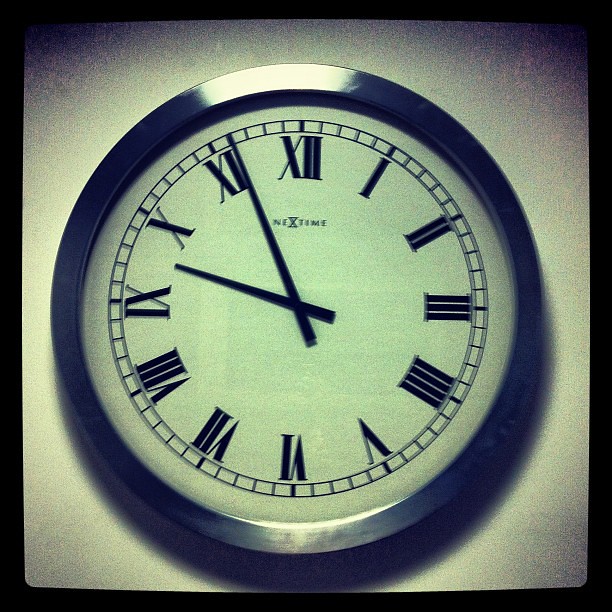This is a detailed photograph of a wall clock with a distinct greenish-blue tinge, likely due to a filter applied to the black and white image. The clock, enclosed in a thin, shiny silver metal frame, is mounted on an off-white, light gray wall. It features a large white face displaying bold black Roman numerals and two hands that indicate the time is approximately 9:56, with the hour hand near the X (10) and the minute hand just past the XI (11). Underneath the 12 o'clock position, the clock brand "NEXTIME" is prominently displayed in capital letters, with the 'X' resembling an hourglass. The wall clock casts a distinct shadow below and slightly to the right on the wall. The photograph itself has a textured, pixelated appearance and is bordered by a black frame, enhancing the depth and vintage feel of the image.